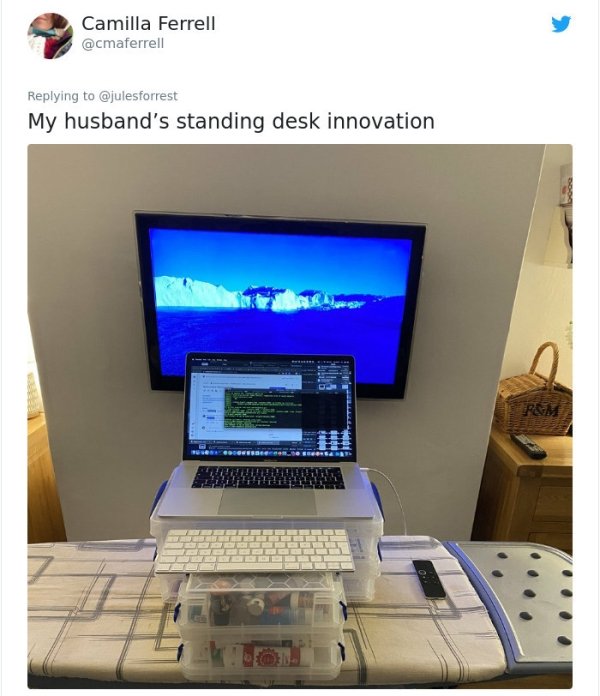In the image, Camilla Farrell (@CMA Farrell) replies to Jules Forrest on Twitter, stating, "my husband's standing desk innovation." Featured prominently is an unconventional standing desk setup, which includes a silver laptop and white keyboard perched atop plastic storage containers, all placed on an ironing board draped with a white cloth and blue trim. Above the setup, a wall-mounted monitor displays a serene scene of icebergs against a blue backdrop. To the right of this setup, a wooden table hosts a wicker basket labeled "R&M" and a TV remote. The background room is modestly lit, with a brown nightstand bearing a black TV box and additional household items scattered about, adding to the improvised and homely vibe of the workspace.